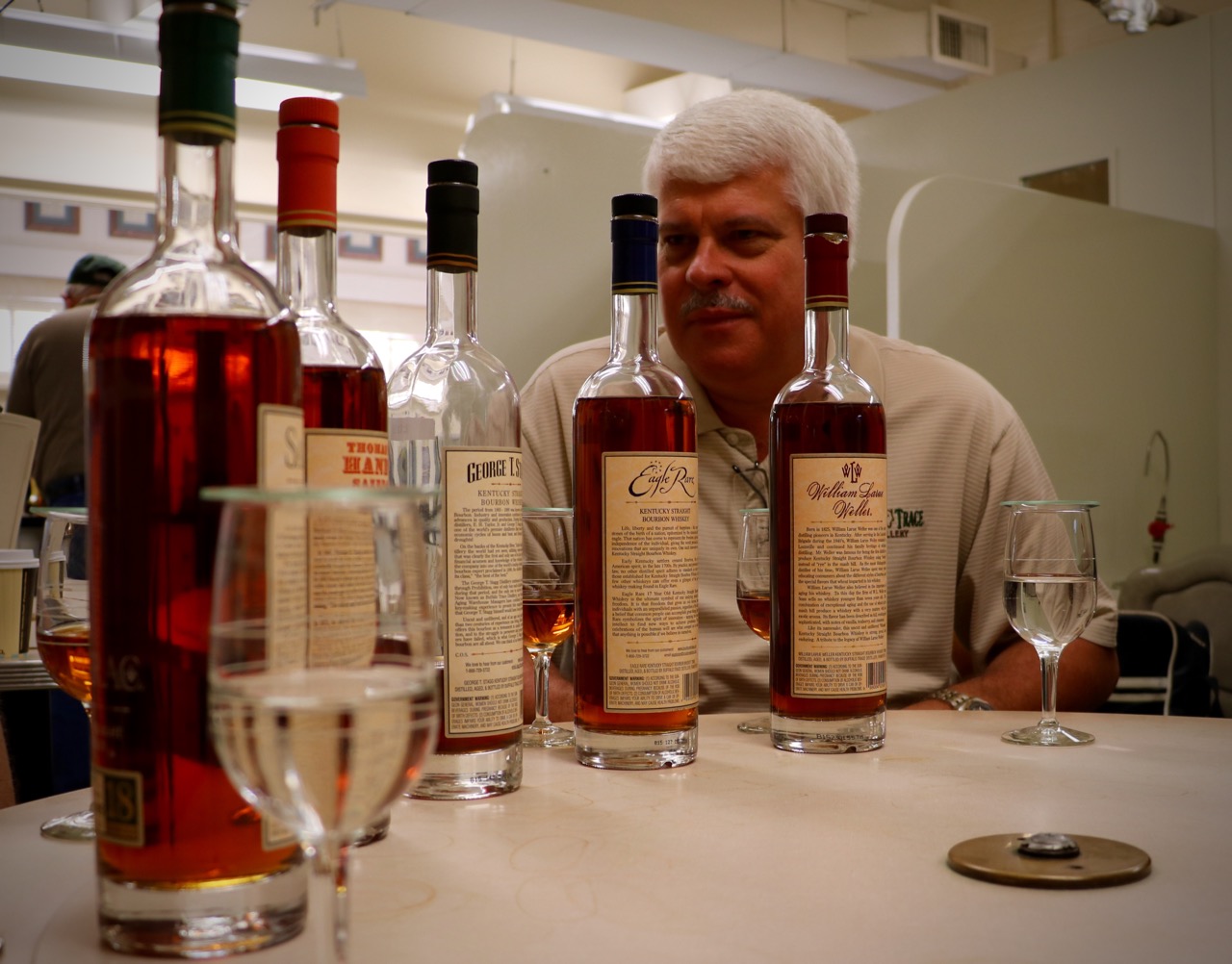In a well-lit restaurant setting, a middle-aged, slightly chubby man with white hair and a salt-and-pepper mustache sits at a light beige tabletop. He is dressed in a short-sleeved white shirt and is surrounded by an assortment of five liquor bottles, each with various levels of dark brown liquid inside. The bottles, adorned with labels featuring intricate designs and small print, have screw-off caps, likely indicating they are whiskey or another type of liquor. In front of him are four glasses: two filled with whiskey or similar liquor, and two half-filled with water or a clear liquid. The man appears to be engaged in a whiskey tasting, listening attentively to someone out of the frame with a focused expression. In the blurry background, another man wearing a cap is visible with his back turned, possibly assisting another group.